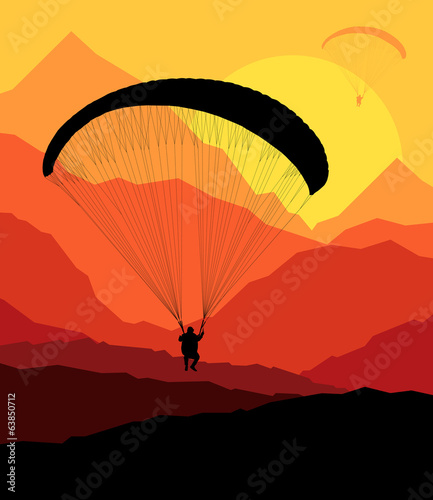This vertical rectangular image is a striking piece of artwork from Adobe Stock (number 63850712) that vividly portrays a colorful parachuting scene. The bottom third of the drawing is dark, representing the ground, transitioning into a vibrant gradient of a mountain range depicted in progressively lighter shades of orange. The mountains, depicted as layered strips resembling construction paper cutouts, ascend from black at the base to maroon, dark red, lighter red, and through to various tones of orange. Above this picturesque range is a radiant sky, with a glowing orange background transitioning to a bright yellow around a setting sun.

In the center of the composition, a black silhouette of a parachutist hangs suspended from a canopy, connected by numerous black strings. Further into the distance, in the upper right corner, a smaller parachutist with a light orange silhouette can be observed, adding depth to the scene. The image captures the essence of a serene and sublime moment, emphasizing the interplay of light and shadow with bold colors and abstract artistry. Along the left edge of the image, there is white text running sideways that reads "Adobe Stock number 63850712," cementing the artwork's uniqueness and source.